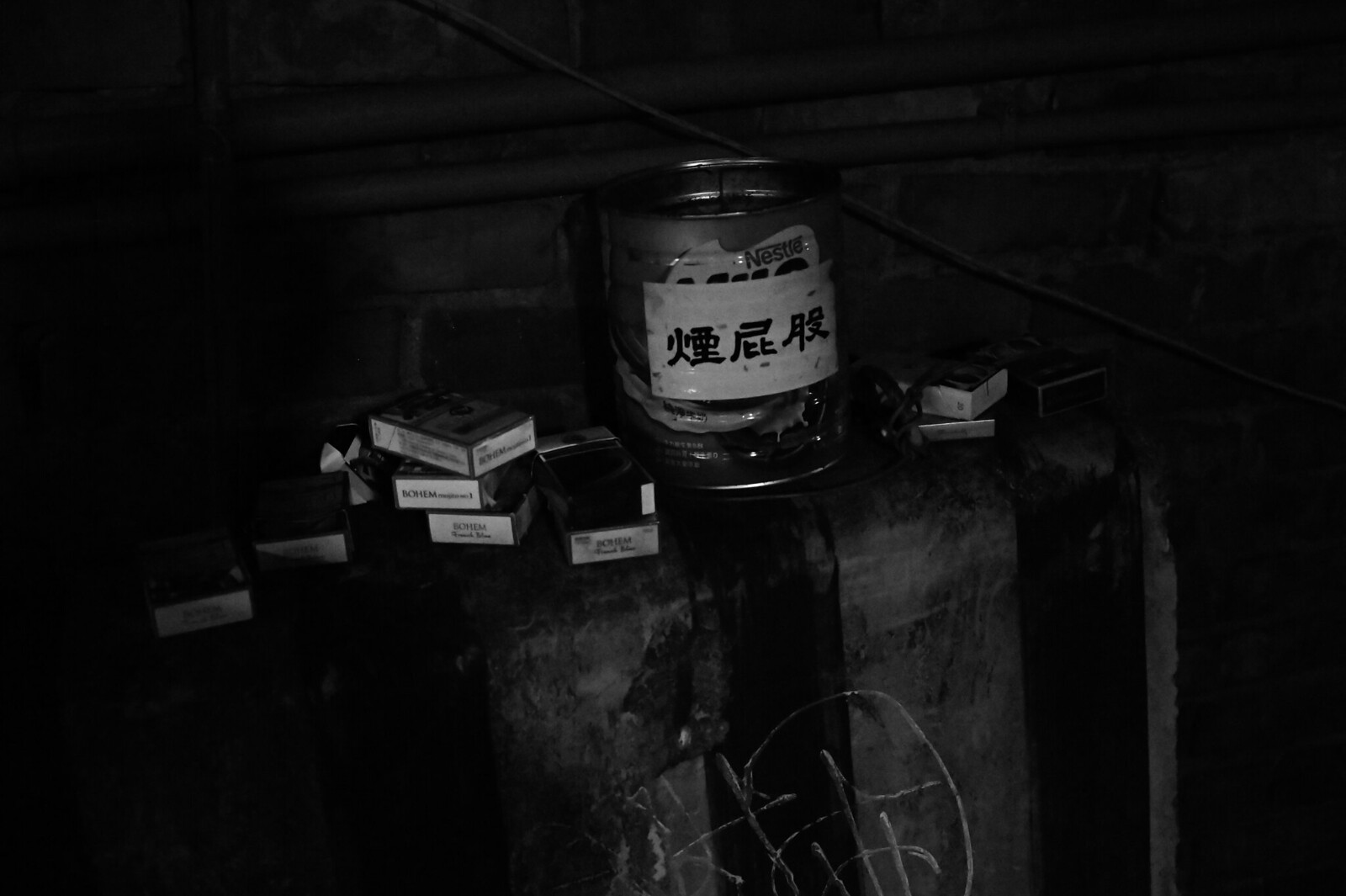This image presents a very dark, almost black-and-white scene that appears to be taken with minimal lighting, making the details hard to discern. At the center of the image is a large jar or tin container prominently featuring a white piece of paper with Japanese or Chinese script, obscuring the original Nestle label. The jar or container is resting on what seems to be a couple of wooden barrels or a dark-covered table with black stripes. Surrounding the jar are several rectangular boxes, some possibly open, with large, capitalized letters "B-O-H-E-M" on them, though the rest of the text is indiscernible. The scene is further obscured by the extremely dark background, potentially a brick wall, which adds to the unclear and mysterious nature of the photograph.